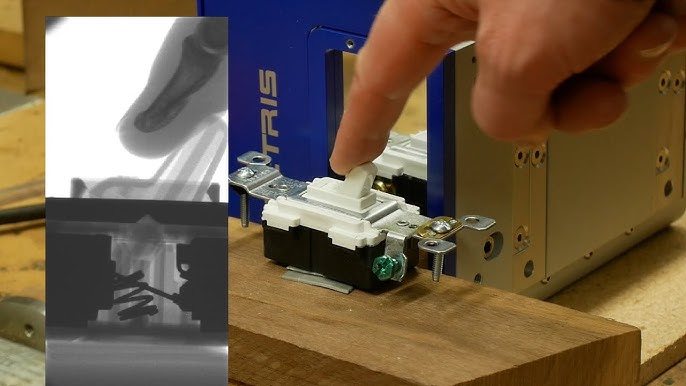The image depicts a detailed science experiment centered around a standard light switch mounted on a wooden block. A human finger is actively pressing the switch into the down position. To the left of this setup are two x-ray images: the top x-ray reveals the intricate skeletal structure of the finger making contact with the light switch, while the bottom x-ray provides an in-depth view of the switch's internal mechanism. Additionally, beside the light switch rests a computer-like device labeled "Altruist," characterized by its blue and metallic gray components, which likely plays a role in capturing or analyzing the experiment's data.